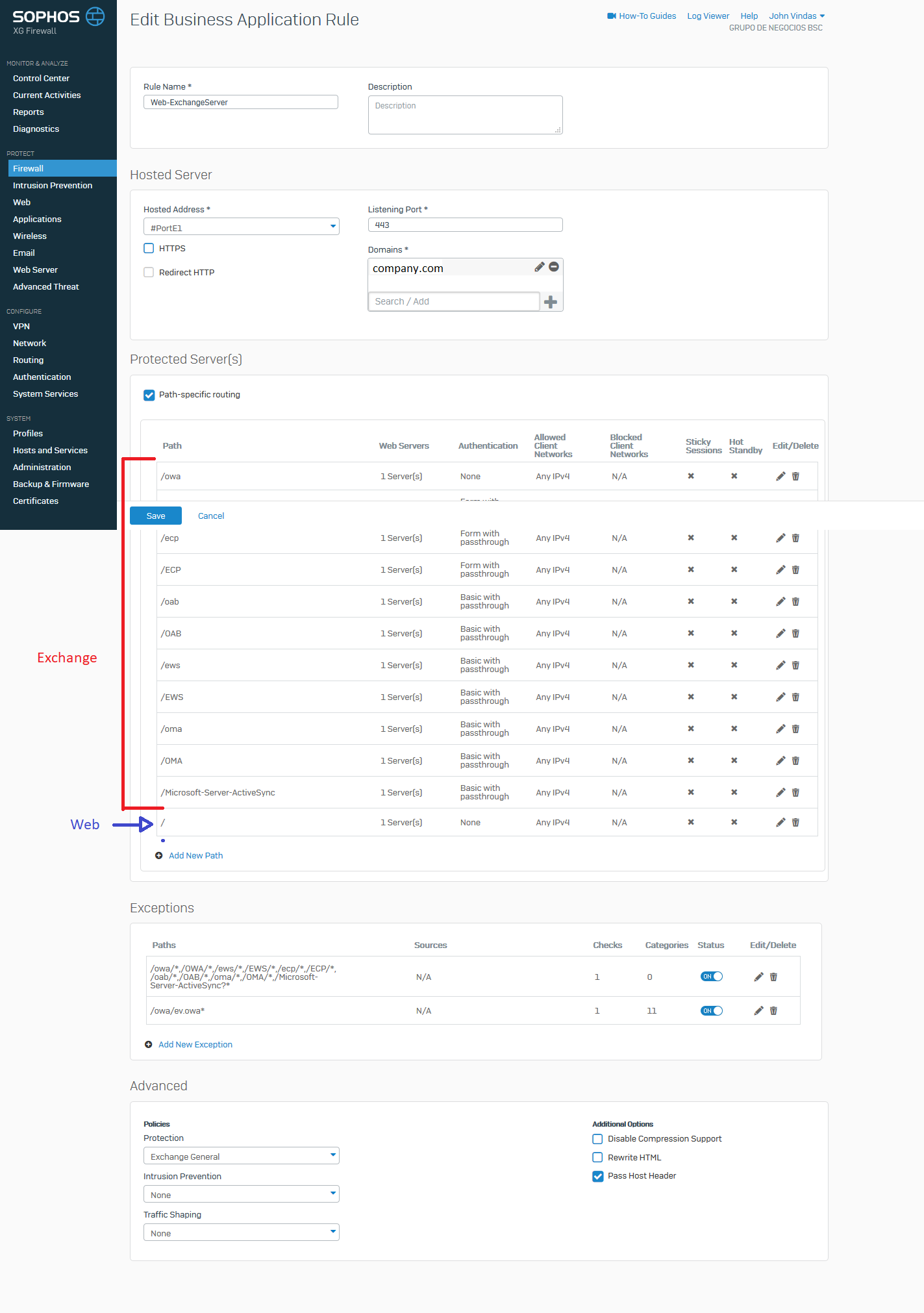On the screen, we see the 'Edit Business Application Rule' page of the Sophos XG Firewall interface, characterized by its user-friendly and detailed layout.

The background is a light gray, providing a neutral setting that doesn't distract from the content. On the left side, a vertical dark blue rectangle captures attention, prominently displaying, in white text, "Sophos XG Firewall" alongside a circular blue emblem. Below this, the sidebar lists various navigation options: Monitor and Analyze, Control Center, Current Activities, Reports, Diagnostics, Protect, Firewall (highlighted within a light blue rectangle), Intrusion Prevention, Web, Applications, Wireless, Email, Web Server, Advanced Threat, Configure, VPN, Network, Routing, Authentication, System Services, System, Profiles, Hosts and Services, Administration, Backup and Firmware, Certificates, allowing for easy access to different sections of the application.

To the right, the main content area starts with the title "Edit Business Application Rule." Beneath this title, a white rectangular box with black text fields begins with "Rule Name" and a specified entry "Web Exchange Server." Adjacent is a description box intended for additional details.

In the upper right corner, we find a small blue camera icon linked to the "How-To Guides," accompanied by options for "Log Viewer," "Help," as well as user information, displaying "John Bendas," and "Grupo de Negocios BSC."

Below the initial form, a larger section labelled "Hosted Server" in black text unfolds. Details within include "Hosted Address," marked as "Hashtag Port E1" via a dropdown menu. Two squares provide options for "HTTPS" and "Redirect HTTP." Beside these, "Listening Port" is depicted, with its value set to "443." The "Domains" section follows, specifying "Company.com."

Further down, another large white square titled "Protected Servers" includes several options and settings. These settings start with a blue box containing a white checkmark and the text "Path-Specific Routing." Below this, various fields and options are listed: Path, Web Servers, Authentication, Allowed Client Networks, Blocked Client Networks, Sticky Sessions, Hot Standby, with options to Edit or Delete.

Below this section, specific entries such as OWA, ECP, OAB, EWS, OMA, and Microsoft Server ActiveSync are displayed successively, each followed by specific configurations, represented in both regular and capitalized text where applicable.

Towards the bottom, a "Save" icon is prominently positioned to ensure changes can be stored. Following this, there are options for adding patches, exceptions, and defining paths, sources, checks, categories, status, with corresponding Edit and Delete actions. "Add New Exception" offers additional customization opportunities.

Finally, at the very bottom, the "Advanced" settings menu presents policies regarding Protection, Exchange General, Intrusion Prevention, Traffic Shaping, additional options like "Disable Compression Support," "Rewrite HTML," and a checkbox for "Pass Host Header," providing comprehensive control over the firewall's behavior and performance.